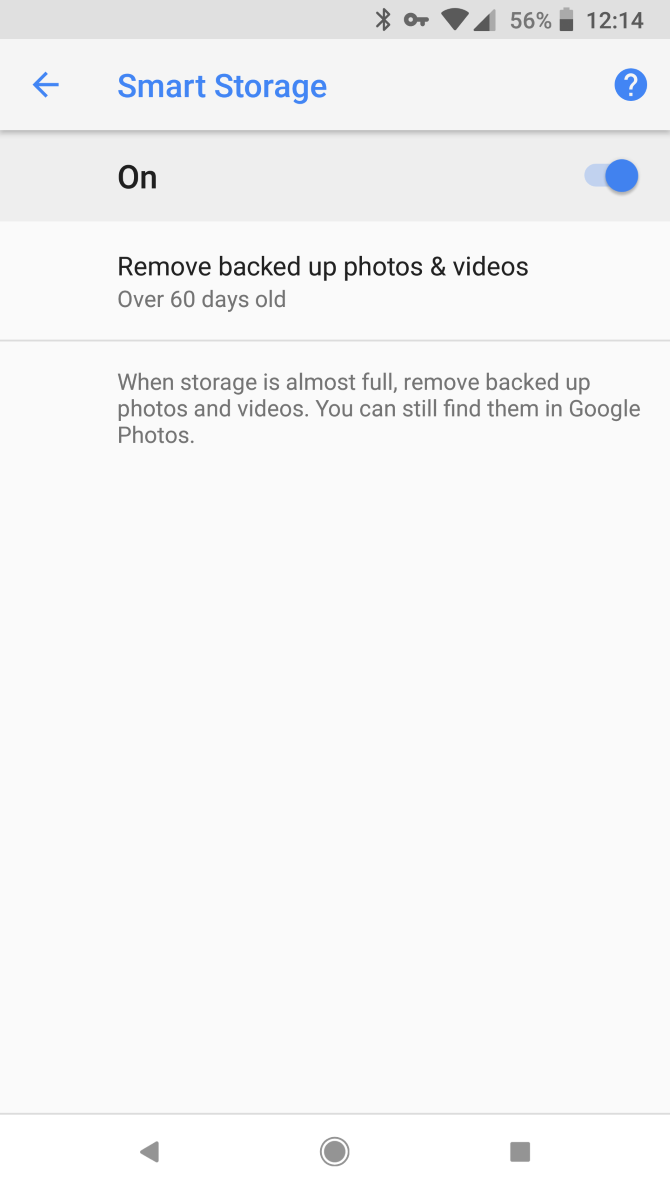The image depicts a smartphone settings page with several informational and toggle elements. At the top of the screen, there is an indicator showing Bluetooth is connected, a key icon, full Wi-Fi connectivity, and a battery level at 56%, all alongside the year 2014. 

Below these indicators, the settings page focuses on storage management. There is blue text labeled "Smart Storage" next to a blue circle containing a white question mark. Underneath this section, there is gray text indicating the feature as "On," accompanied by a toggle switch. 

The options provided include "Remove backed up photos and videos over 60 days old," with a horizontal divider separating it from additional text. This additional text explains that "When storage is almost full, remove backed up photos and videos" and reassures that users can still find these items in Google Photos. Another horizontal line follows this information, and various shapes—a sideways triangle, a circle, and a square—all appear in gray.

The entire settings page has a clean, white background, making the text and icons stand out clearly.